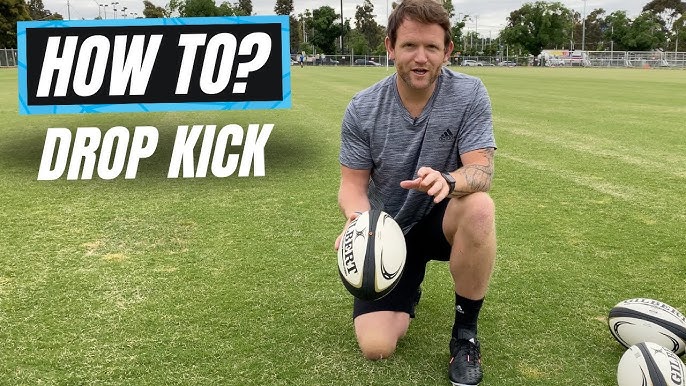The image depicts a Caucasian male in his early 40s with short, brown hair and a slight beard concentrated around his chin, suggesting a five o'clock shadow. He is dressed in a short-sleeved Adidas shirt, primarily dark blue with some white, identifiable by the Adidas logo on the top right. He holds a rugby ball in his right hand, which is predominantly white, adorned with black and yellow markings, and labeled "Gilbert" in black, serif font. The background features a gradient of light blue at the top transitioning to black at the bottom. To his left, the text "HOW TO DROPKICK" is prominently displayed in all-caps white font. The man appears from the waist up, with his left hand outstretched. Behind him, partially obscured, is additional text in off-white, hinting at the letters "Y-B-R-I-C-K-S" at the top right of the image.